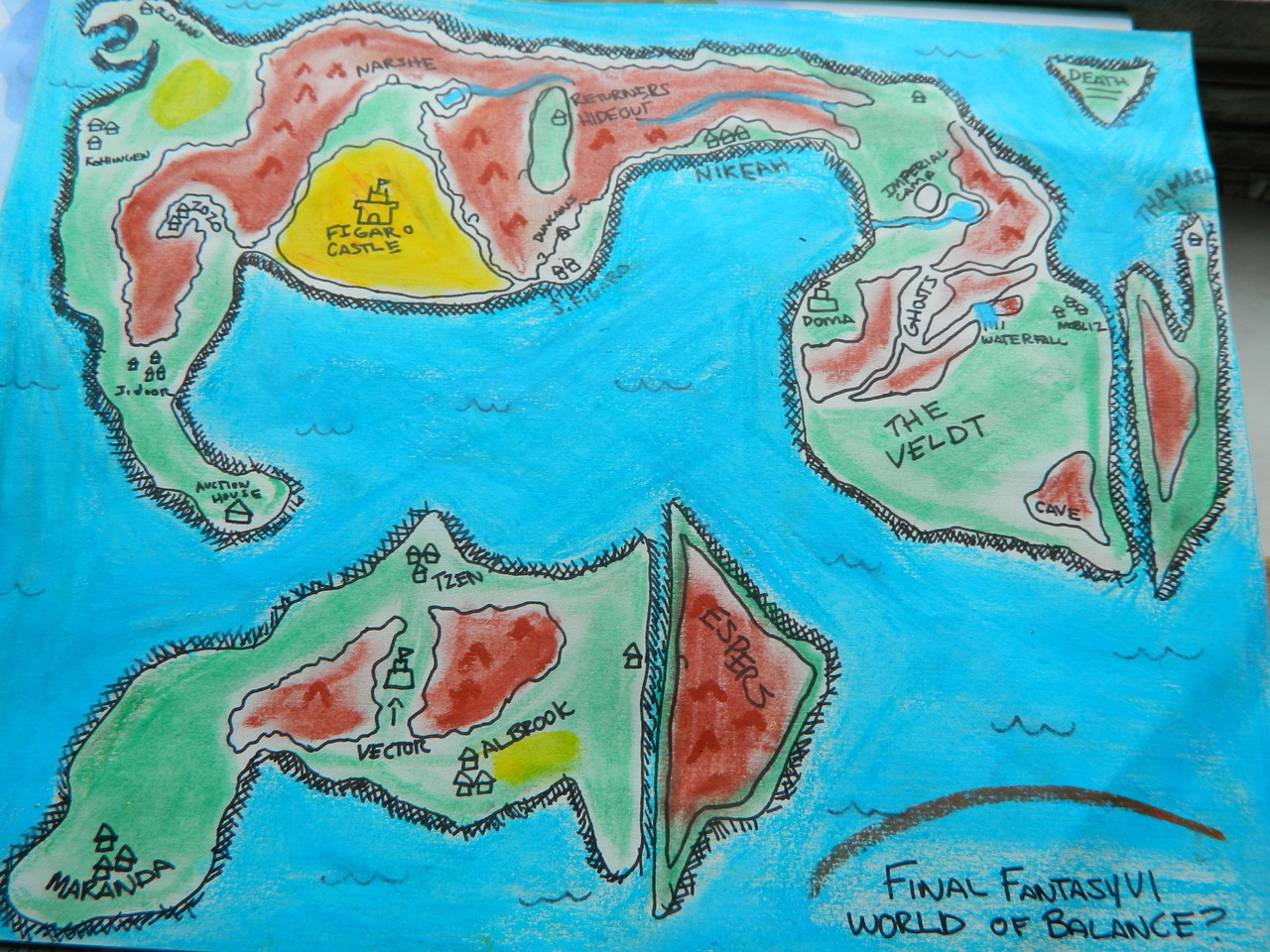This is a meticulously hand-drawn map of the Final Fantasy VI World of Balance, rendered with crayon or colored pencil. In the bottom right corner, the text "Final Fantasy VI World of Balance?" is inscribed in capital letters and penned in black ink. The map features two main land masses, with the larger, deformed island occupying the top half of the image. This top region includes prominent landmarks such as Figaro Castle, mountains, Narshe, and the Returner's Hideout on the left, while the right side houses locations like the Veldt, Doma, the Imperial Camp, and a Waterfall. 

The lower part of the map contains a smaller landmass featuring a mountain designated for Espers and several notable towns like Vector, Albrook, and Miranda positioned in the bottom left corner. Further distinguishing highlights include an island labeled 'Espers' to the right of the smaller landmass and an upside-down triangular island in the top right corner marked 'Death'. The map is encircled by a vividly colored blue ocean, detailed with wave marks, amplifying its artistic flair. The use of red, yellow, green, blue, and black colors contributes to the map's vibrant and detailed appearance, indicating various locations and terrain features, all labeled in clear capital letters.